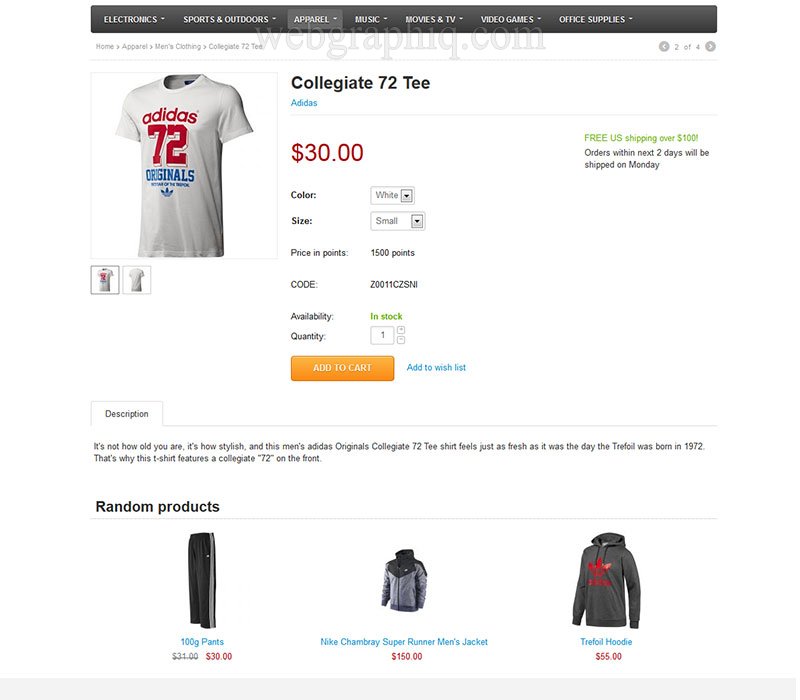A detailed web page from a shopping site is displayed on a computer screen. The site has a professional layout with a grayish-black navigation bar at the top, showcasing various clickable tabs. A watermark reading "WebGraphIQ.com" is subtly visible. In the top-left corner of the page, there is an image of a white t-shirt with the text "Adidas 72 Originals" prominently displayed. This t-shirt, labeled as "Collegiate 72T," is priced at $30, with the price written in maroon, while other text is in black. An orange "Add to Cart" button is positioned below the price.

The website's background is primarily white, with certain elements highlighted in a lime-green color. The text "Free U.S. shipping over $100" stands out in this green color. Under the "Availability" section, the word "in-stock" is also highlighted in green. Below this, a small box contains a product description, and further down the page, there is a section titled "Random Products" separated by a gray line.

This section features additional items, including a pair of pants, a jacket, and a hoodie, all of which appear to be from the Adidas brand, as suggested by the visible logo on the hoodie. A light gray bar stretches across the very bottom of the page, completing the layout.